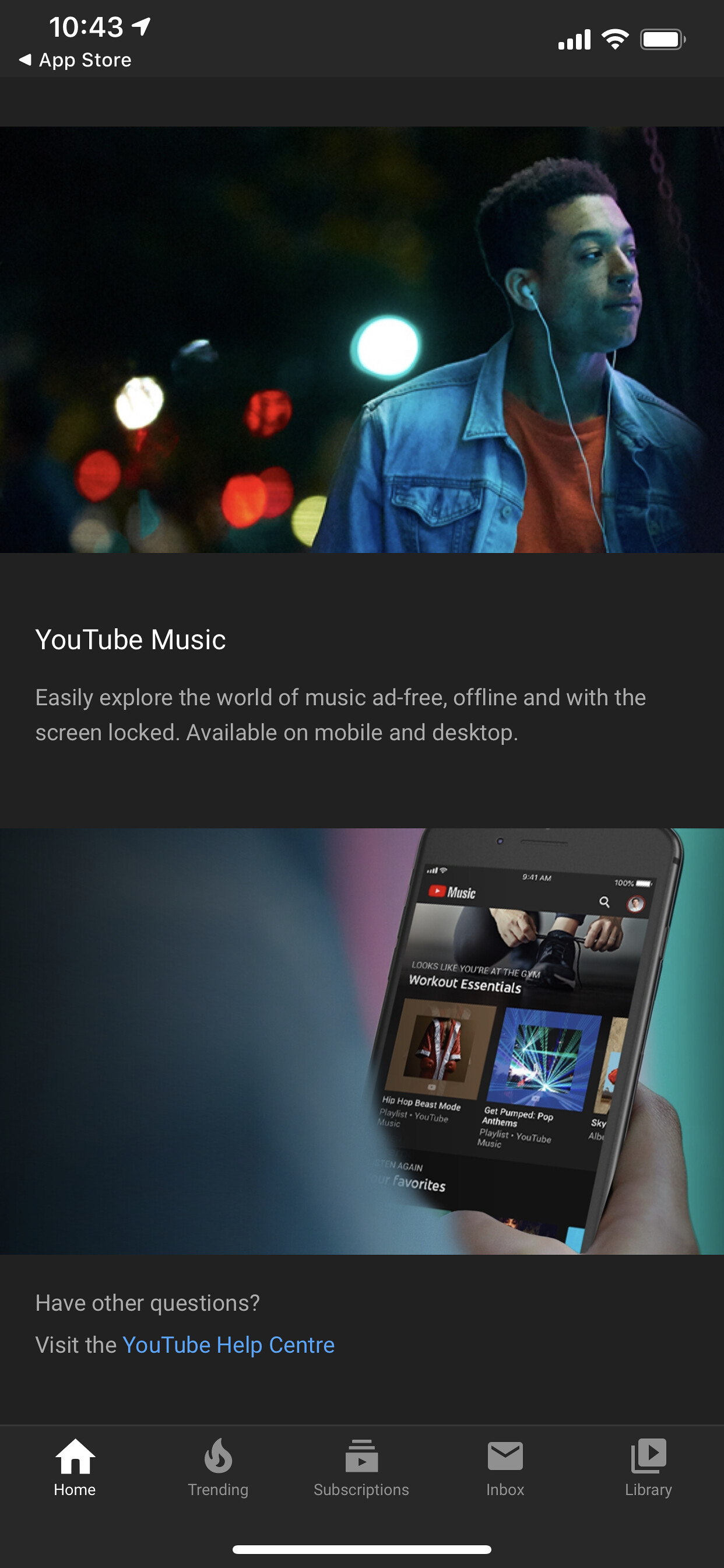This advertisement showcases a person enjoying music, emphasizing the features of the YouTube Music app. 

At the top of the advertisement, the number "1043" is prominently displayed, followed by smaller text that reads "Available on the Backyarrow App Store." Below this, the main headline "YouTube Music" stands out, accompanied by a description: "Easily explore the world of ad-free music, offline playback, and background listening with the screen locked. Available on mobile and desktop."

The upper section of the advertisement features an image of a young man gazing thoughtfully into the distance. He is wearing a denim button-up shirt and headphones, visually representing the immersive music experience.

In the lower part of the advertisement, there is a close-up of a smartphone screen displaying the YouTube Music app interface. The screen showcases two album covers, highlighting the app's user-friendly appearance. Below the smartphone image, a prompt reads: “Have other questions? Visit the YouTube Help Center.”

At the bottom, a dark banner contains navigation options for the app: "Home," "Trending," "Subscriptions," "Inbox," and "Library." The text on the banner is vibrant white, providing a sharp contrast against the dark background, which is a theme consistent throughout the advertisement for visual emphasis.